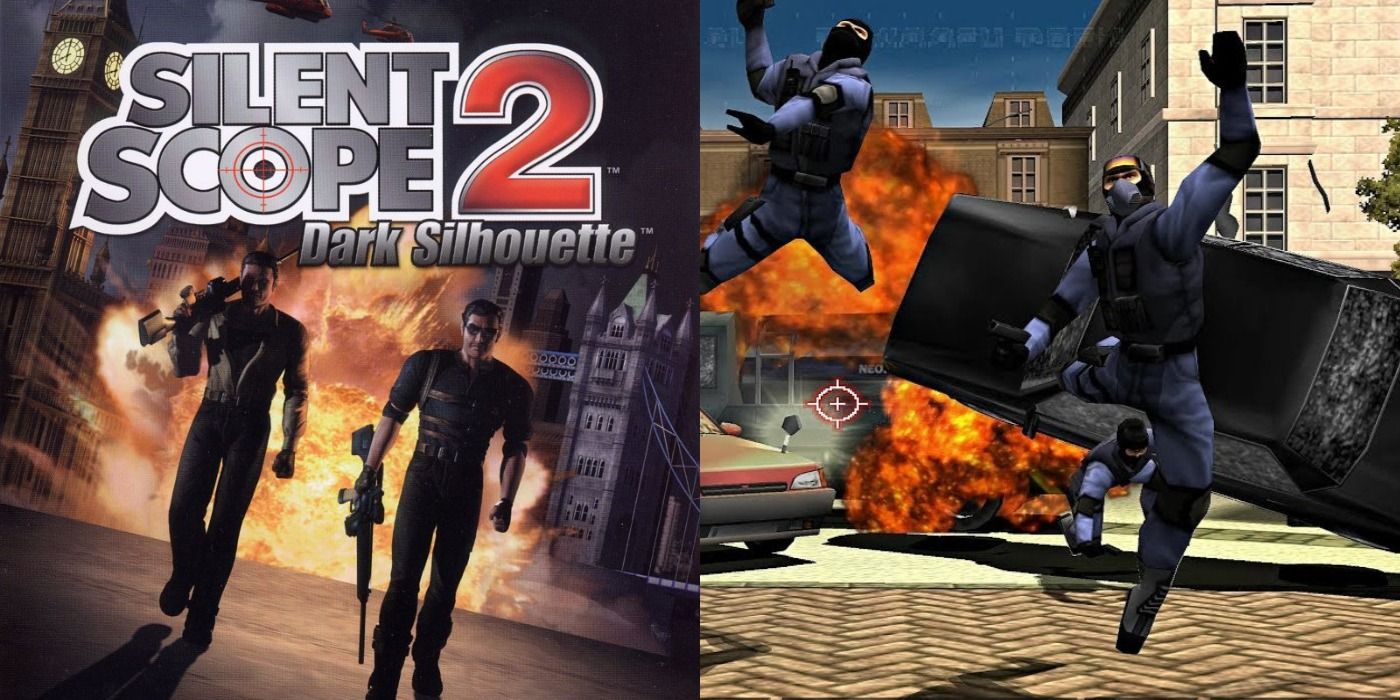The image is an oblong-shaped poster, seemingly for a movie or a video game cover, composed of two distinct sections. On the left side, against a white background, large gray letters spell out "Silent Scope," with the "O" featuring a red bullseye, followed by the number "2" in bold red-blue. Below this title, "Dark Silhouette" is written in a striking silver.

The left section depicts two men, likely mercenaries or soldiers, dressed in black. The man on the left sports a tan leather jacket and black pants, carrying a sharp-shooting rifle slung over his shoulder. The man on the right wears a black sweater with a shoulder harness, black sunglasses, and an assault rifle at the ready. They are shown walking away from a massive explosion, with iconic London landmarks like the London Bridge and Big Ben Tower in the background.

The right section of the poster presents an intense city scene. Another explosion occurs, sending the two men—possibly the same duo from the left image—flying through the air. One man is seen near a car, which is also caught in the explosion, flipping dramatically in the background. A crosshair reticle appears on the left side of this part, possibly hinting at sniper gameplay elements.

Overall, the poster combines elements of destruction and urban warfare with an air of cinematic or gaming excitement, unified under the title "Silent Scope 2: Dark Silhouette."